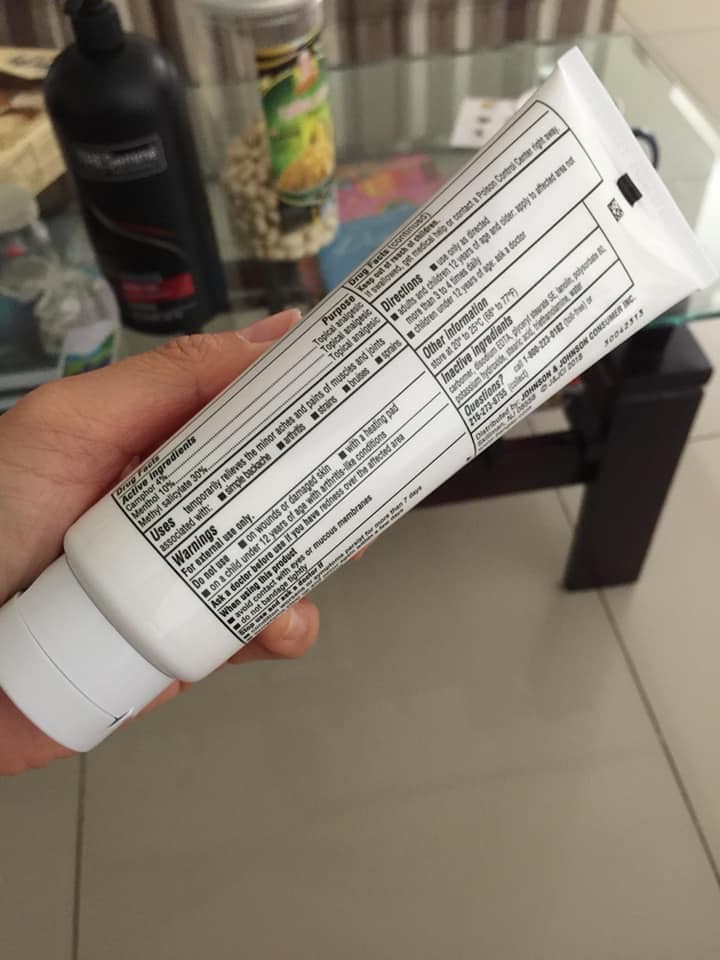In the image, a person is holding a tube of medication, which is used for temporarily relieving minor aches and pains of muscles and joints, commonly associated with ailments like arthritis. The scene is set on a glass table, which is raised above a wooden table with a brown finish. On the right side, there is a jar with a green label containing white nuts. Adjacent to it, there is a bottle that likely contains shampoo, recognizable by its familiar shape and a red emblem resembling a monument. To the left of the shampoo bottle, there is a bag of an unidentified item. The background features metallic elements, adding a slight industrial feel to the setting, while the floor beneath is adorned with white tiles.